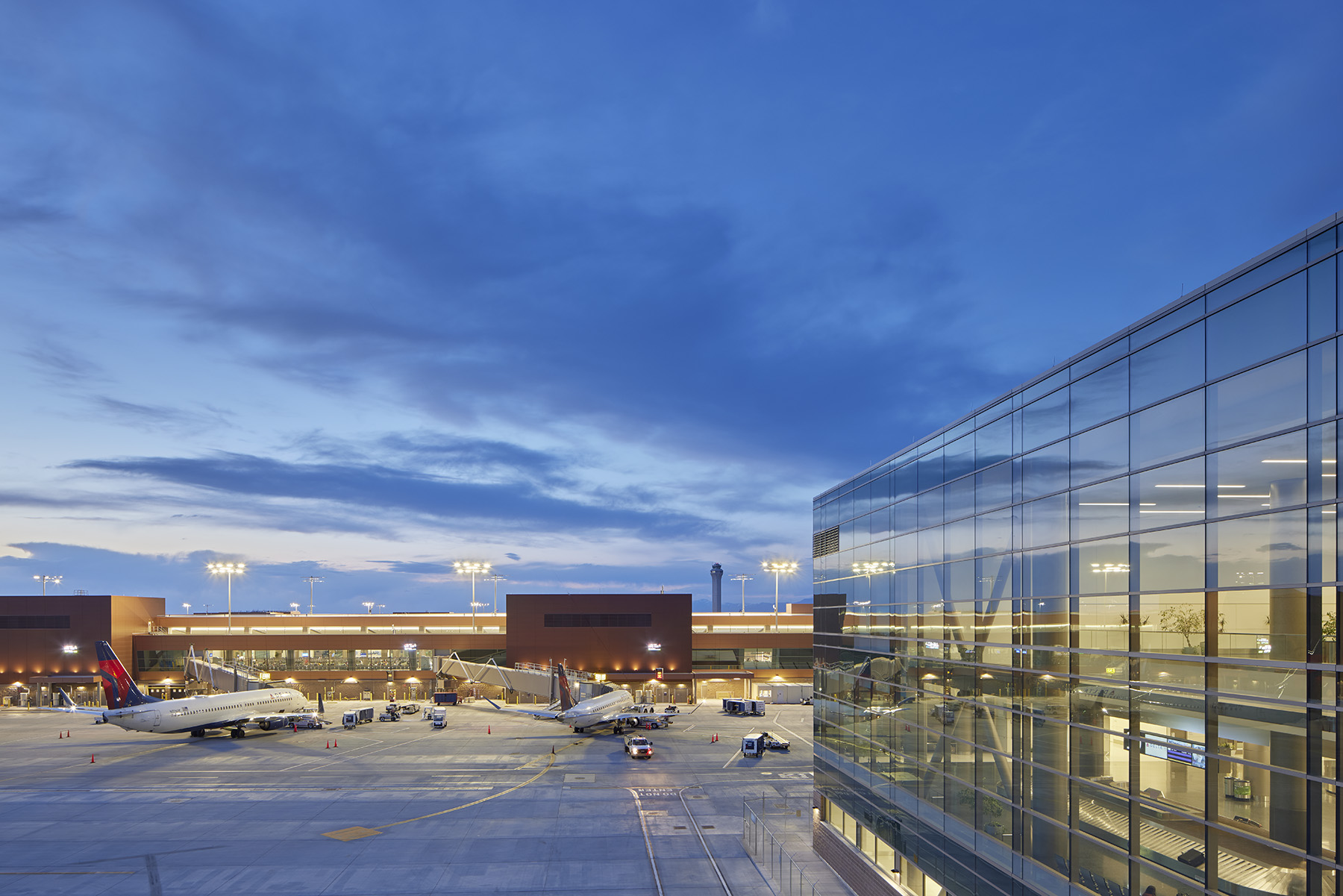In this detailed photograph of an airport taken at dusk, the sky is a rich, dark blue with scattered clouds, transitioning into the deeper hues of evening while bathed in a subtle light from the setting sun. The airport below glows warmly with yellow lights as night approaches, providing an illuminated contrast against the encroaching darkness.

To the right, an intriguing glass and iron structure stands prominent, offering a clear view inside where a luggage belt loops with bags, the interior appearing empty and isolated. This building, possibly housing offices or operational staff, features a grid-like pattern on its façade, adding architectural interest. Further in the background, a long, low brick building stretches across the scene, adorned with lights on its roof that shine brightly onto the runway, delineating the various functional areas of the airport.

Two airplanes, identifiable by their Delta logos, are docked at the airport. Entry walkways connect them to the terminals, indicating ongoing loading or unloading activities. The runway is populated with various service vehicles, including luggage carts and miniature traffic cones, scattered around the vicinity. Although the scene is bustling with vehicular activity, it retains a serene and calm ambiance. The distant silhouette of the air traffic control tower reinforces the expansive and comprehensive layout of this tranquil, yet bustling airport at dusk.